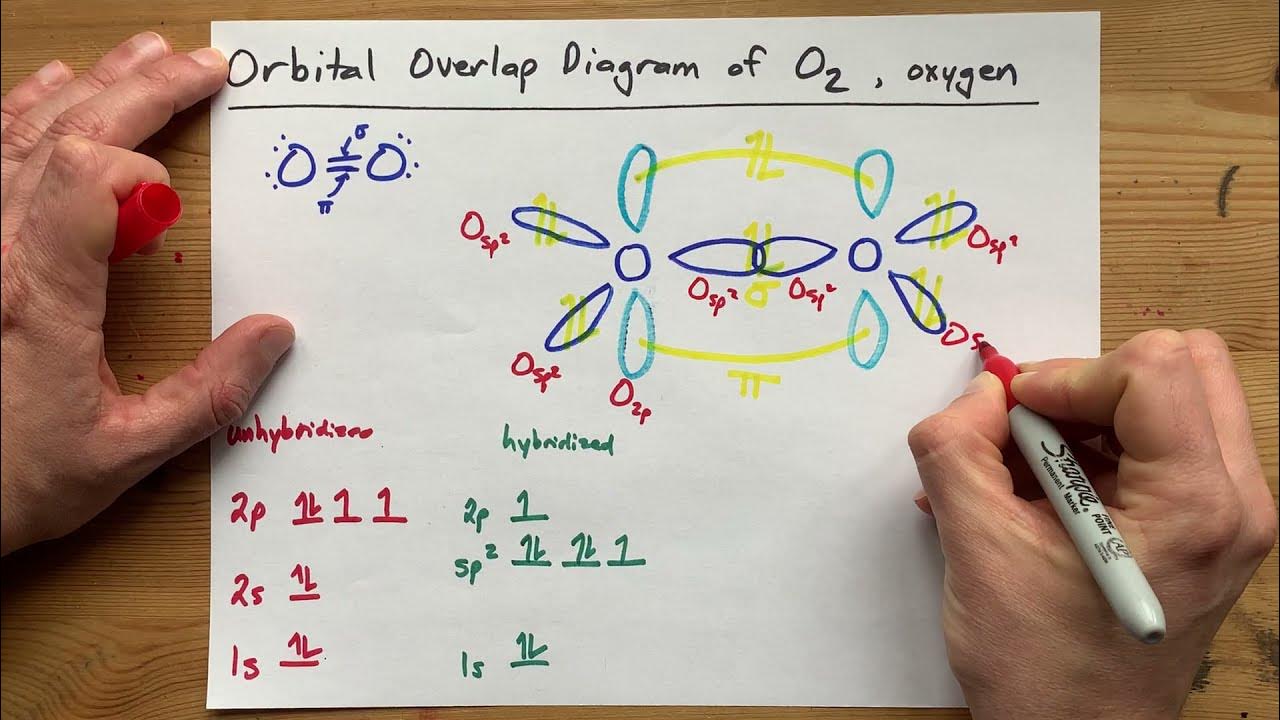A horizontally aligned photograph captures a white-skinned individual drawing a scientific diagram with a red Sharpie marker on a white office paper sheet, placed on a light wooden table with visible wood grain. With the left hand holding the page in place at the upper left corner and gripping the red marker cap with a curled index finger, the right hand actively writes. The paper prominently features the label "Orbital Overlap Diagram of O2 Oxygen" along the top, rendered in black marker. The intricate drawing, comprising abstract interconnected shapes, is meticulously colored with shades of yellow, light blue, dark blue, red, and green. The lower left section of the sheet displays numerical data and mathematical formulas in columns: one labeled "unhybridized" in red and the other "hybridized" in green. The entirety of the visually rich setup emphasizes the detailed scientific work in progress, enhanced by the multi-colored annotations and diagrammatic specificity.